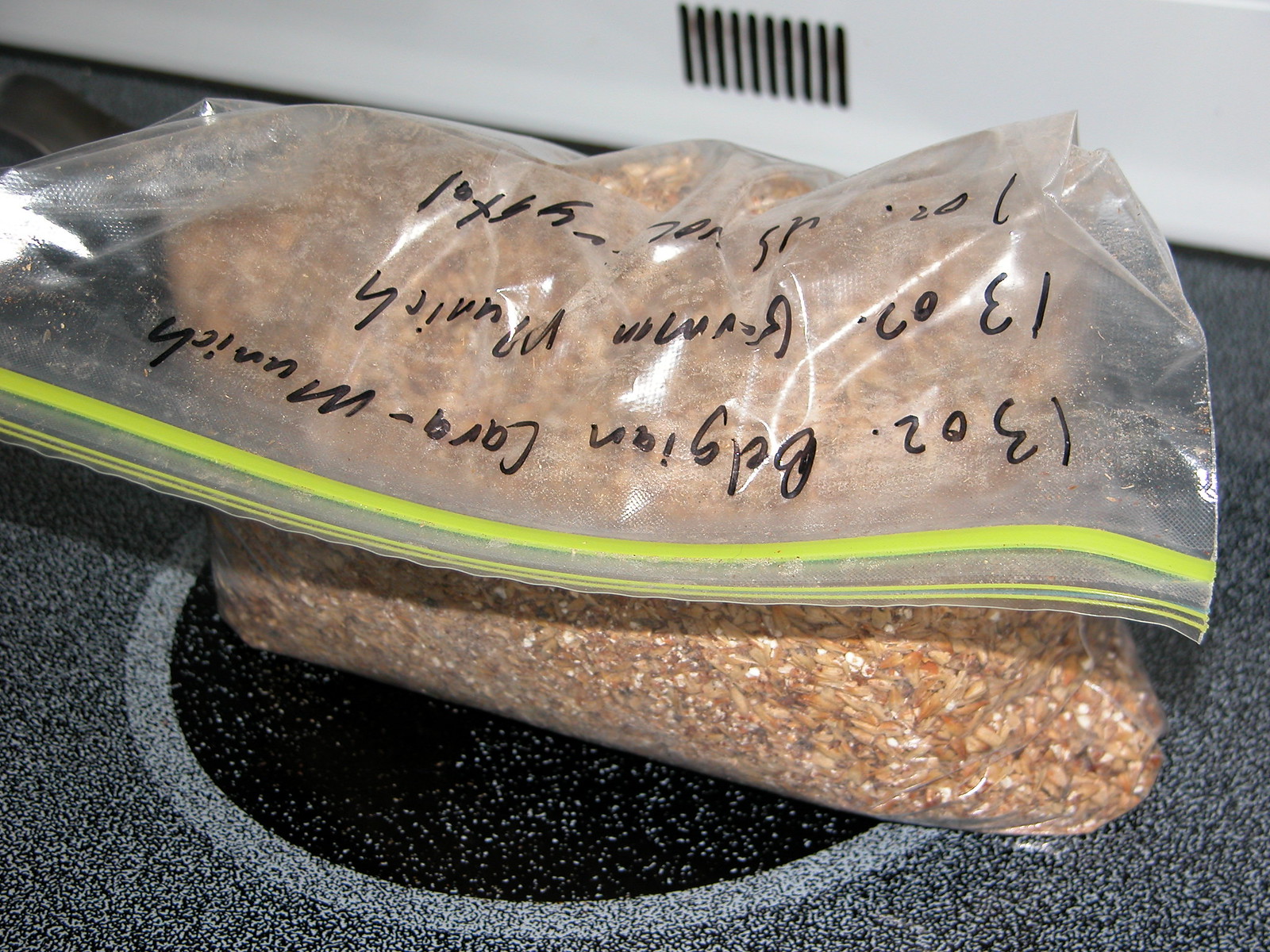The image depicts a large, square photograph focused on an electric stovetop with a white background wall featuring vertical vents at the top. Resting on one of the speckled gray and white burners is a clear Ziploc bag with yellow stripes at the top. The bag is filled with tiny brown seeds, some mixed with white. The top of the Ziploc bag is folded over and has writing in black marker, which is partially upside down. The legible text appears to read "1302 Belgian" and "Munich", although the exact details of the writing are difficult to decipher.